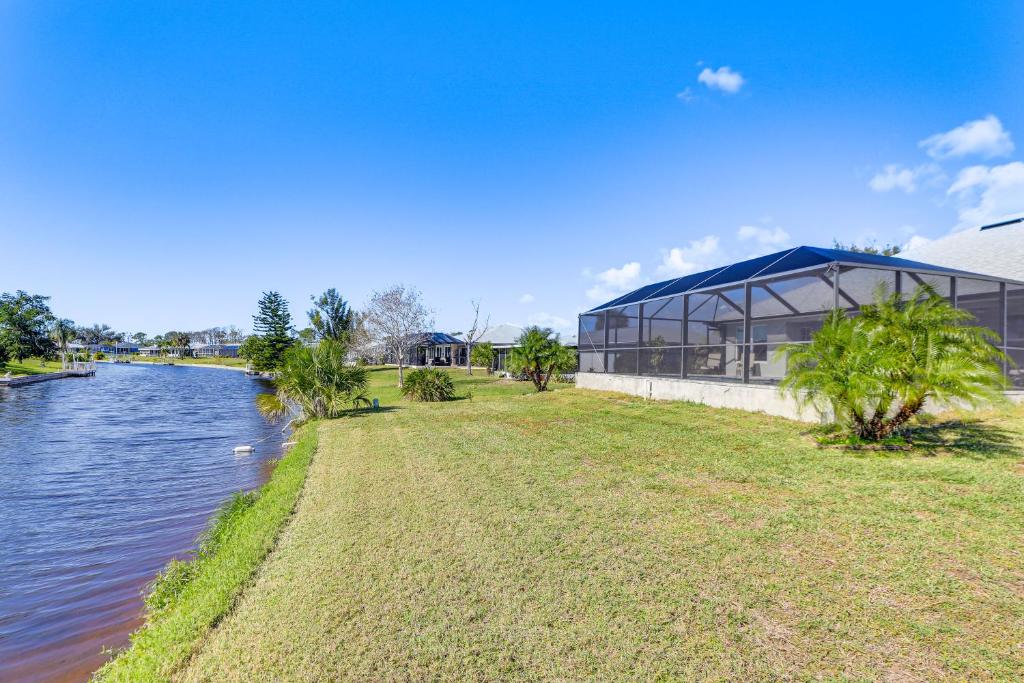The photograph captures a serene backyard scene in a rectangular landscape orientation. Dominating the left side of the image, a small canal or lake with dark brown water winds its way from the bottom left corner toward the horizon in the center. The water is bordered by taller green grass along the banks. Above, the light blue sky gradually fades to white as it meets the horizon, scattered with puffy white clouds in the top right corner.

Centrally placed in the lower section of the image, a neatly trimmed grassy yard is punctuated by a few small, spaced-apart palm trees and bushes. On the right side, a single-story, white-painted house with a large covered patio or screened pool area extends into the scene. The patio is framed with large black-outlined panels and features a dark blue roof. Adjacent to the pool area, a stand of three short palm trees adds to the tropical ambiance. Further into the distance, additional houses are partially hidden by trees and shrubs, contributing to the idyllic and tranquil setting. The overall impression is one of peaceful, suburban outdoor living, captured with photographic realism.